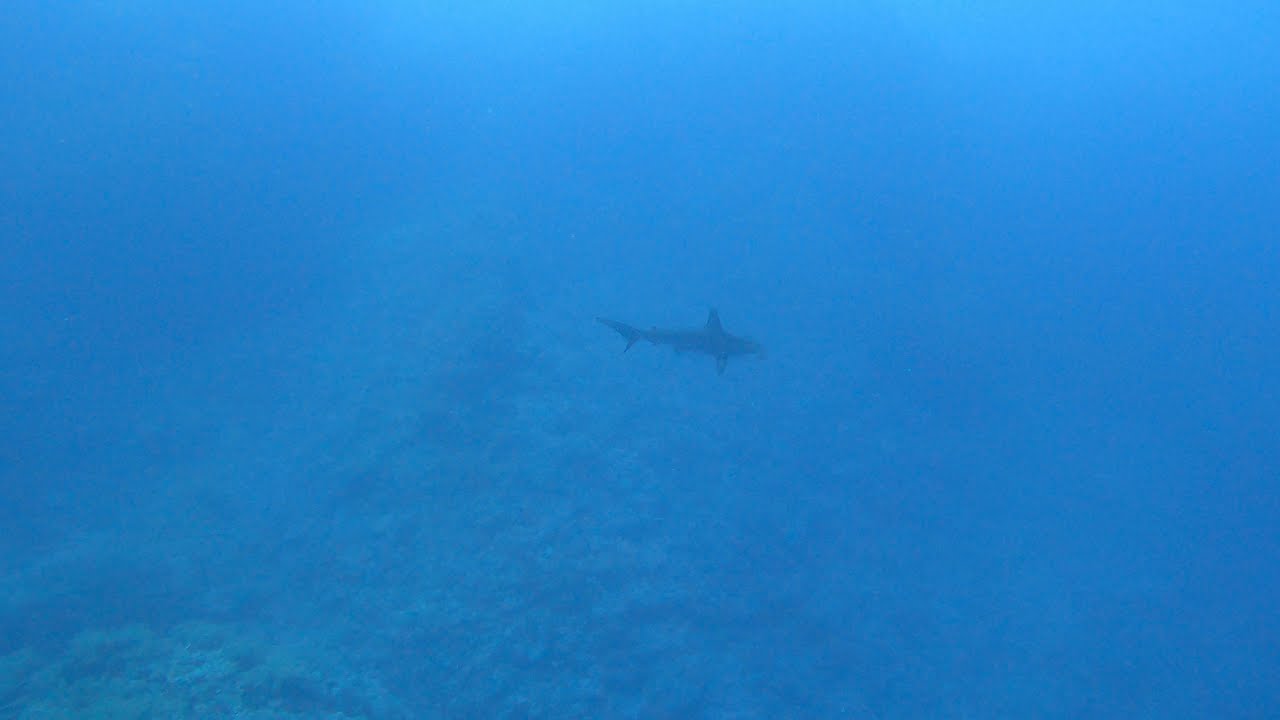This underwater photograph captures a scene in the ocean where the water is a light blue, slightly murky and opaque, making it difficult to see fine details. In the center of the image, a dark, blurry silhouette of a shark is visible, swimming amidst the cloudy water. The shark's shape, fins, and tail can be discerned, though not in sharp detail. Below the shark, towards the bottom of the photo, there are indistinct textures suggesting the presence of a coral reef or some kind of sea growth. The image is dominated by various shades of blue, creating a serene yet mysterious underwater ambiance.